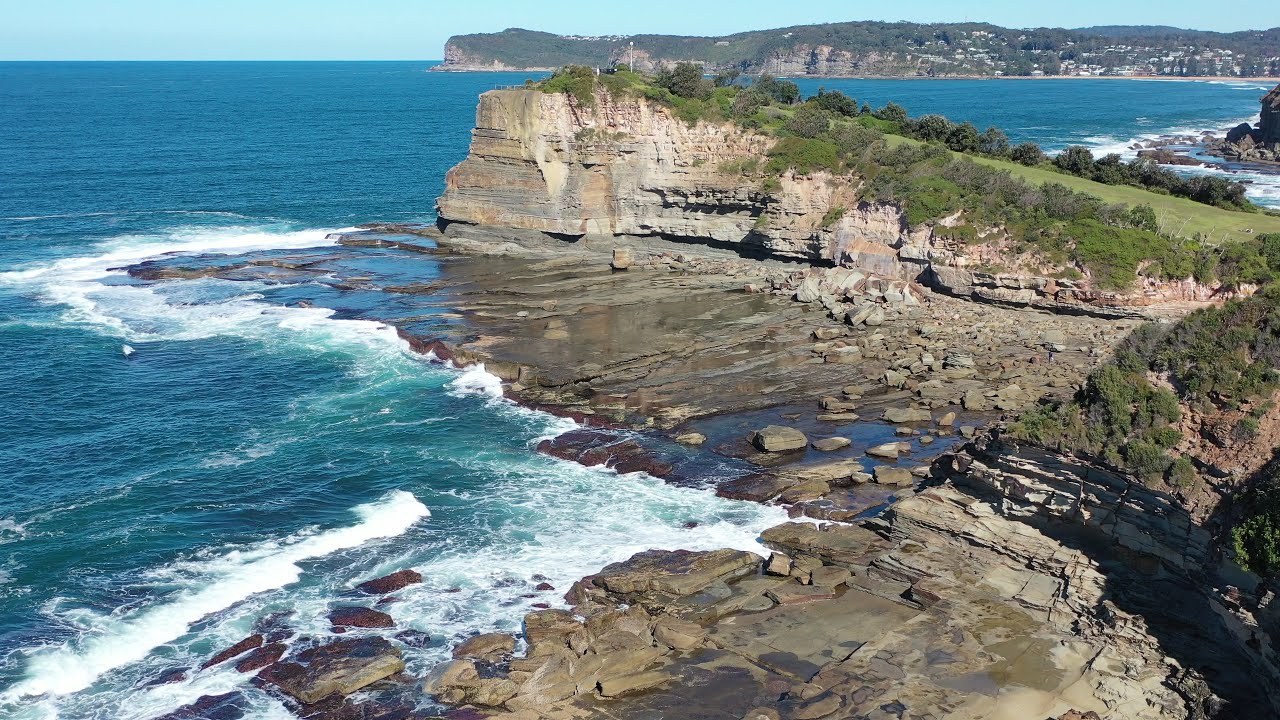This photograph captures a stunning coastal landscape in a landscape format layout. The left side of the image is dominated by a vibrant, dark blue ocean with white crested waves crashing onto the rocky terrain. The water creates a frothy effect at the forefront of the bottom middle of the image. The coastline, characterized by sheer cliffs and a variety of rock formations—from square-shaped to very flat rocks—zigzags in and out, creating a dramatic meeting point between land and sea.

The right half of the photograph showcases the rocky terrain, gradually elevating into lush greenery. The cliffs are adorned with patches of green grass, bushes, and trees. At the very top of the image, a blue sky stretches across the horizon, adding to the serene yet dynamic nature of the scene. In the far distance, the faint outline of buildings suggests the presence of a town. The overall focus of the image is the collision of the ocean's waves against the rocky coast and the subsequent transition into a verdant, elevated landscape.